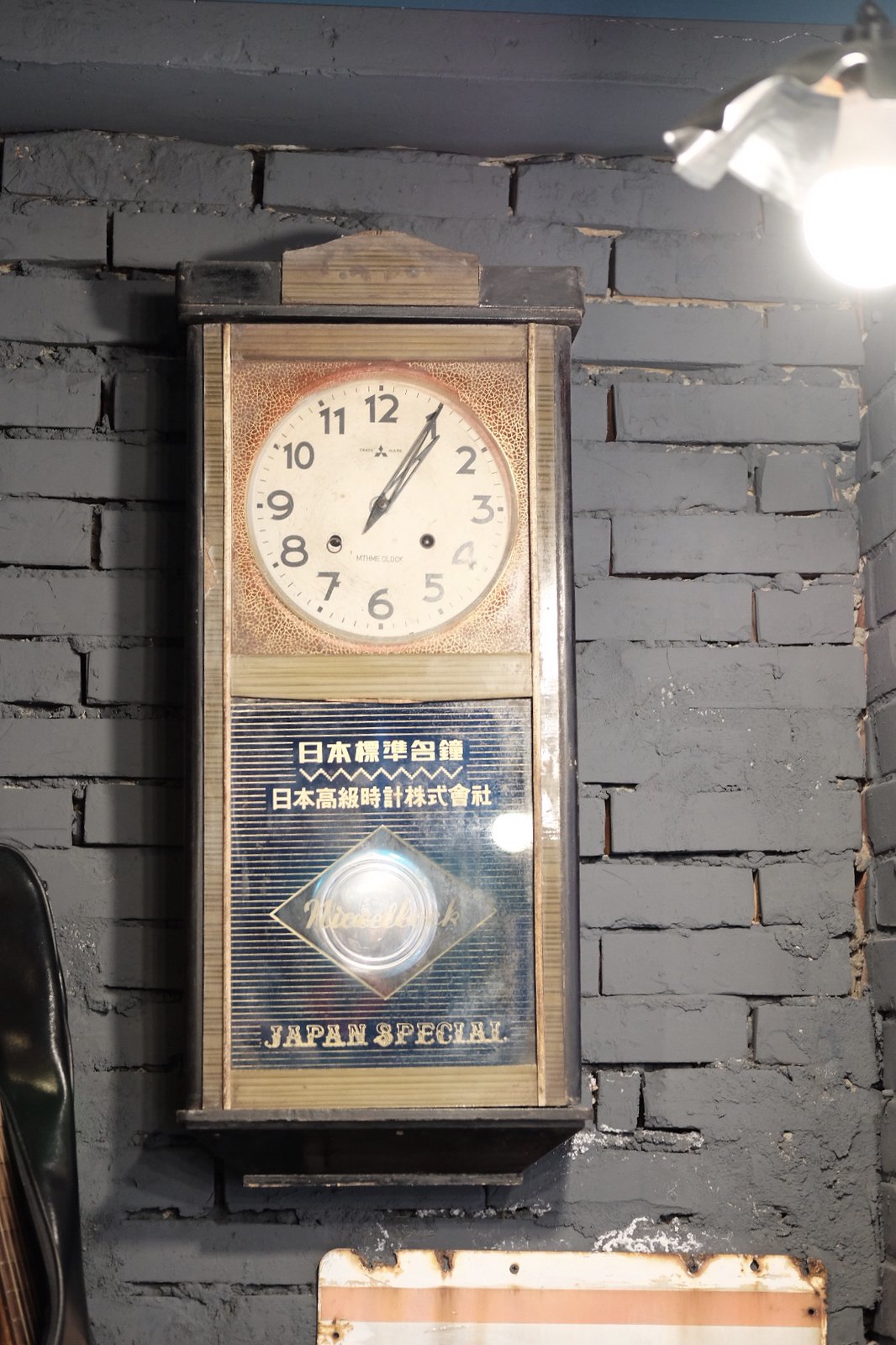The image depicts a slate-gray brick wall, where the bricks are meticulously arranged, but the grout lines vary in coverage, giving it a rugged appearance. The upper right corner of the wall is illuminated by a bright white light. Mounted prominently on the wall is a unique rectangular wall clock, crafted from oak-colored wood and trimmed with darker black wood. The clock face features standard numerals, with its long, brown hands pointing to 1:05. Above the clock face, delicate Japanese calligraphy is displayed, while below it, the phrases "Japan Special" and another Japanese inscription can be seen. Beneath the clock, the top of a white table is visible, adorned with a pink rectangle. The setting evokes a basement-like atmosphere, with the clock subtly coated in dust and seeming in need of cleaning.